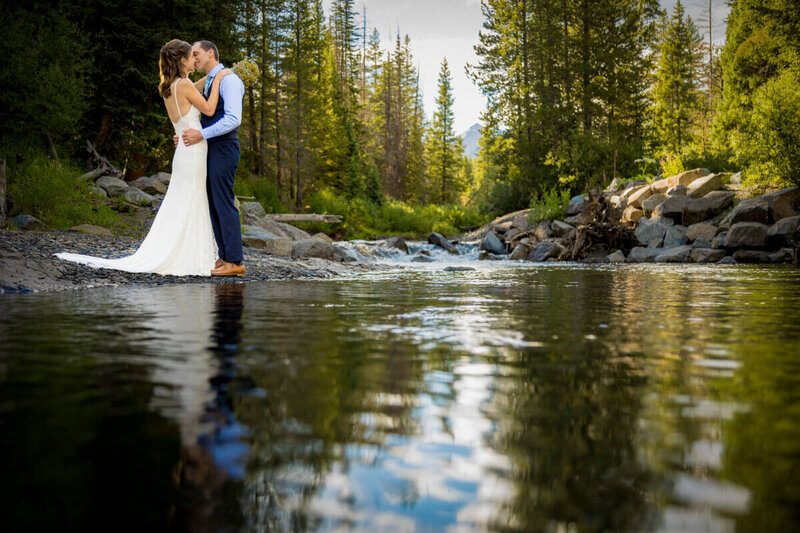The image captures an intimate and picturesque moment from a wedding photo shoot, featuring a white couple standing by the edge of a tranquil river or stream. The bride, a thin woman with shoulder-length brown hair, is dressed in an elegant, long cream wedding gown with spaghetti straps and an open back. Her groom, who is slightly balding with brown hair, wears a chic yet casual dark blue suit paired with a light blue long-sleeved shirt and brown loafers. They are embracing and sharing a kiss, with the groom gently holding the bride's waist.

The photograph is taken from a low angle, near the still water's edge, almost at the water level, giving prominence to the serene river that flows towards the camera. The background showcases a breathtaking natural landscape, including a dense, piney forest and a majestic mountain range peeking through the trees. Stones are scattered along the riverbanks, framing the couple perfectly in the top left corner of the composition. This beautifully captured moment reflects the serene and romantic ambiance of their special day.